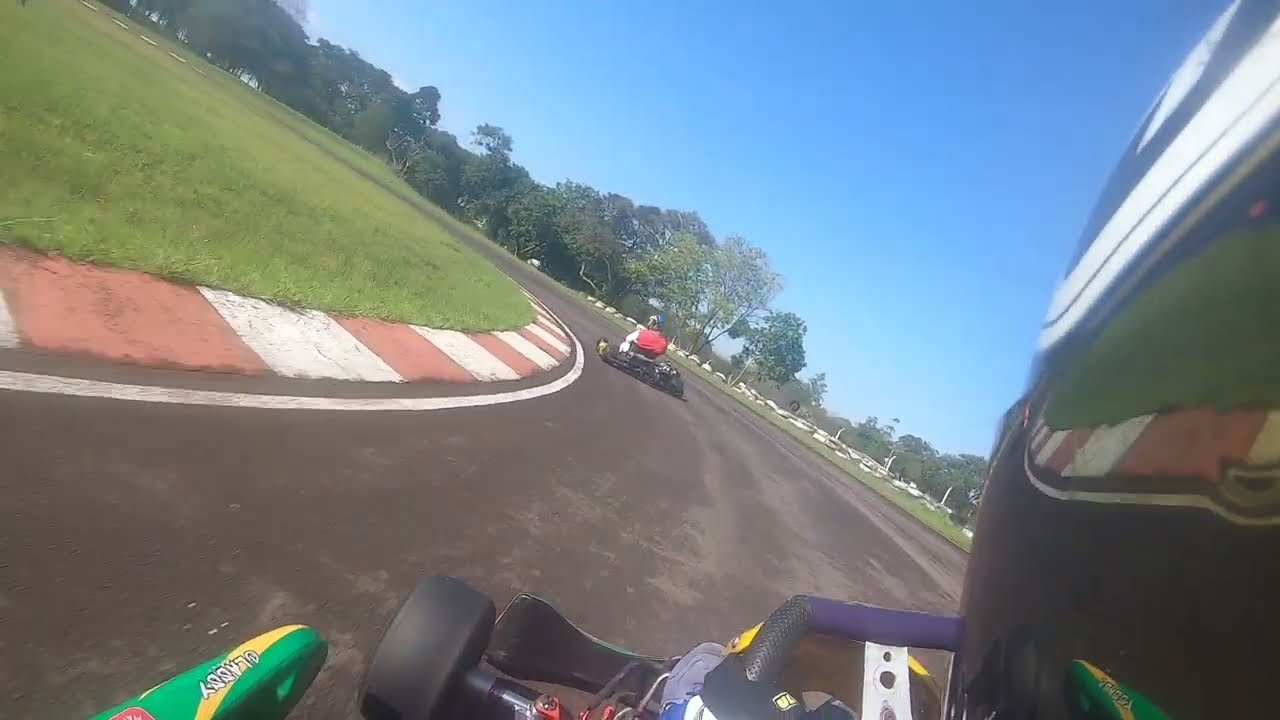The image captures dynamic outdoor GoPro footage of a go-kart race. On the right side, a segment of a driver's helmet is visible, revealing part of a colorful go-kart with shades of black, green, and purple. The driver is navigating a curved section of the asphalt track, which is outlined with alternating white and red squares. Just ahead, another go-kart is seen, driven by an individual maneuvering around the bend. Surrounding the track, fields of grass span both sides, and in the distance, a line of trees stretches across the horizon. The bright blue sky forms a vivid backdrop, while white tires serve as bumpers along the track edges, enhancing the vividness and detail of the race scene.